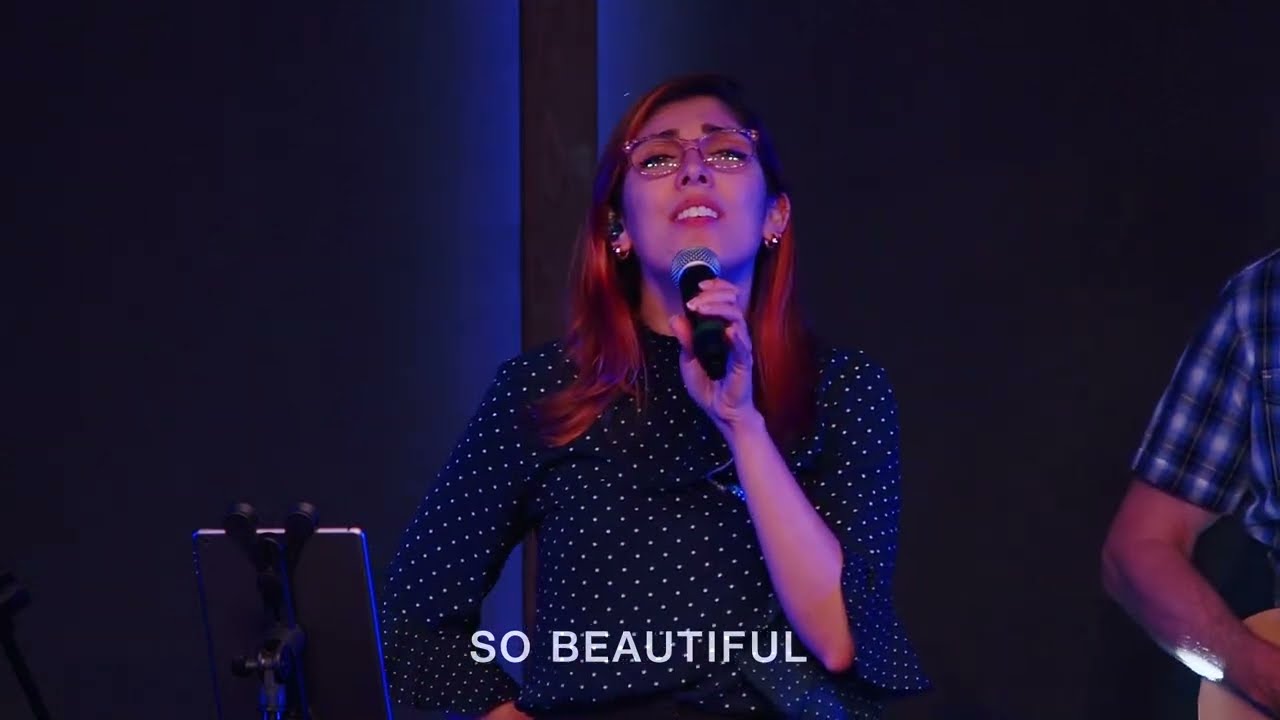The photograph captures a live music performance, showcasing a female singer as the central focus against a black background illuminated with subtle blue stage lighting. Standing at the center, the singer has shoulder-length hair that transitions from a brownish hue at the top to a reddish shade at the ends. She sports cat-eye glasses and gold hoop earrings, with her mouth open mid-song, revealing her top teeth. She's dressed in a navy blue or black top adorned with small white polka dots. In her left hand (positioned on the right side of the image) she holds a microphone, and she has a mounted eye pad to aid with the lyrics. To her right, the visible arm of a guitar player shows he is wearing a blue, black, and white plaid short-sleeved shirt. At the bottom of the photograph, the text "so beautiful" is clearly displayed.